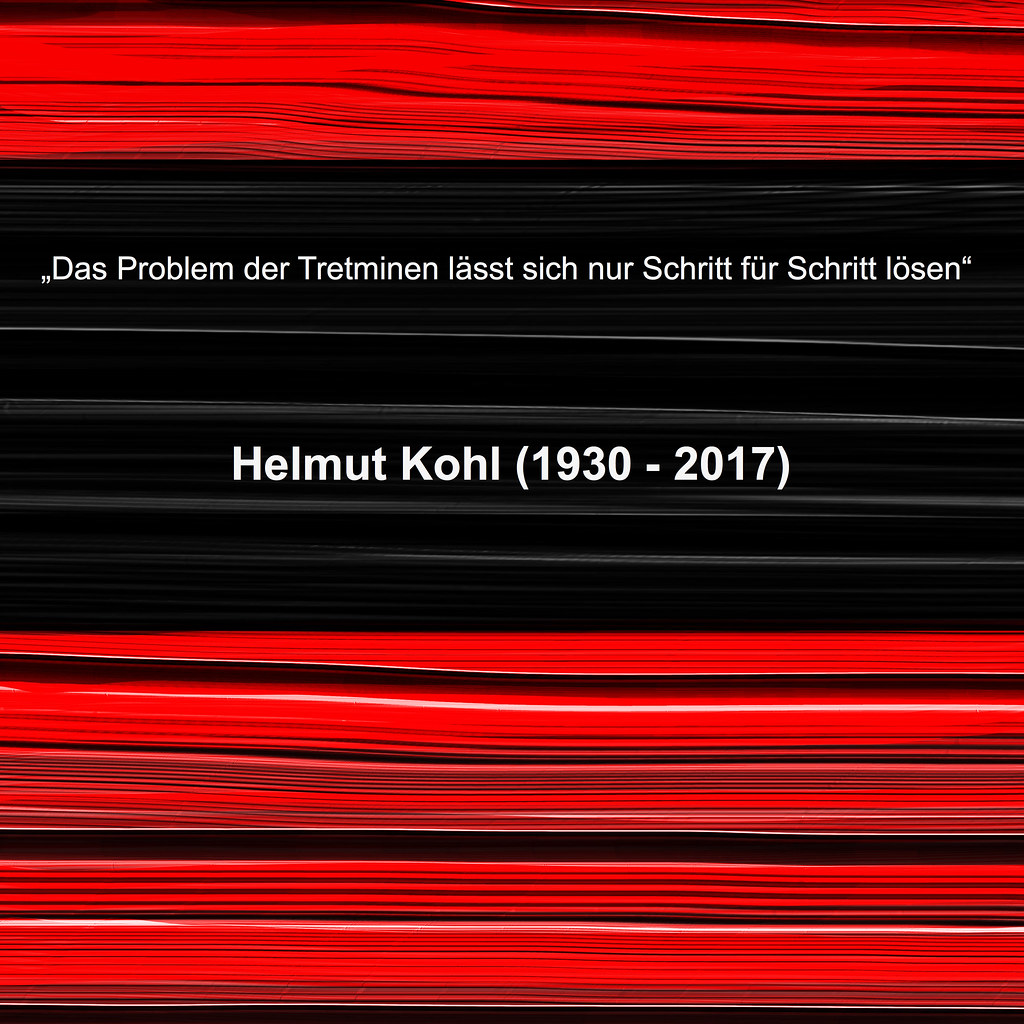This photograph captures a memorial piece for Helmut Kohl, who lived from 1930 to 2017. The memorial features a striking composition of red, black, and white colors. The focal point is a quote in German: "Das Problem der Terrormenten Last Sitz nur Schritt für Schritt lossen," displayed at the top middle section, written in white text against a predominantly black background. Directly below the quote, in a larger white font, is the name Helmut Kohl and the years of his life, 1930-2017. The background incorporates streaky lines that traverse the image, creating an intricate pattern of horizontal and wavy lines. These lines crisscross over the red sections at the top and bottom of the piece, framing the central black area housing the text. The overall size of the memorial piece is approximately four by four, and while the material is uncertain, it appears to be painted or printed, emphasizing its solemn and artistic tribute.